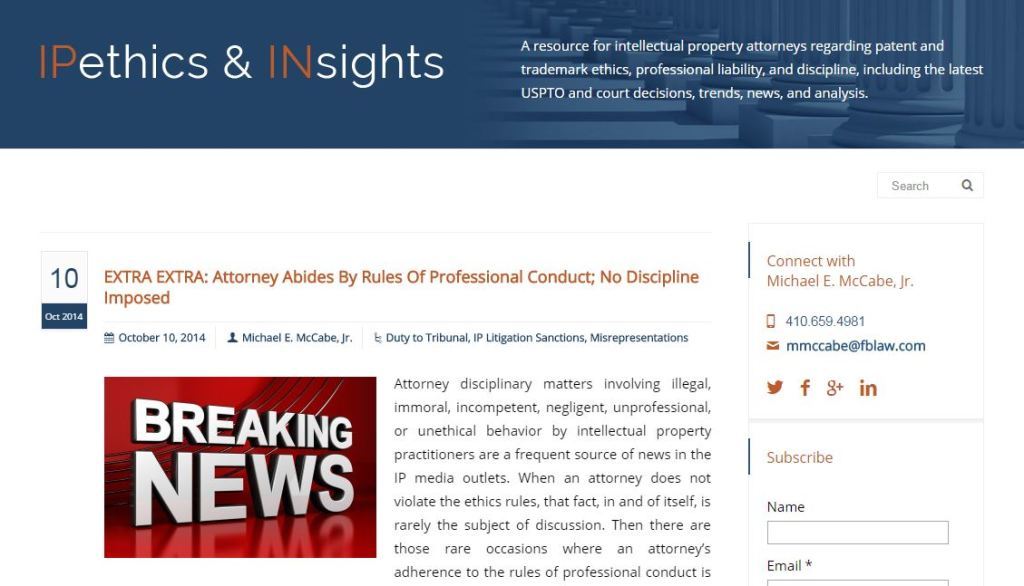### Detailed Descriptive Caption:

The image features a structured layout with a variety of text colors and elements. On the left-hand side, a teal background is presented with nearly the entire phrase "IP" visible. The central portion of the image prominently displays the word "Ethics" in white, accompanied by a hand symbol. Following this, there appears to be partial text "IN," succeeded by the clear, white text "CITES."

Beneath this, a comprehensive description in white reads: "A resource for intellectual property attorneys regarding patent and trademark ethics, personal liability, and discipline, including the latest USPTO and court decisions, trends, news, and analysis."

A noticeable section of white space below this text features a search box with the word "search" and a gray magnifying glass icon.

The left side also contains important information in orange text, stating: "Extra. Extra attorney advised by rules of professional conduct, no discipline imposed."

A thin gray line separates this from additional text in teal that reads: "October 10th, November 2014, Michael E. McCabe, Jr."

Another set of text details various topics such as "duty to tribunal IP," "litigation sanctions," and "misrepresentations," followed by a black-colored description discussing attorney disciplinary matters involving unlawful, immoral, incompetent, negligent, unprofessional, and unethical behavior by intellectual property practitioners. It also emphasizes the discussion generated when an attorney does not violate the ethics rules. However, it trails off, indicating a cutoff point.

On the opposite side, in orange text, the phrase "Connect with Michael E. McCabe, Jr." is displayed. In teal blue, the text "MMCCABFBLaw.com" concludes the visible elements of the image.